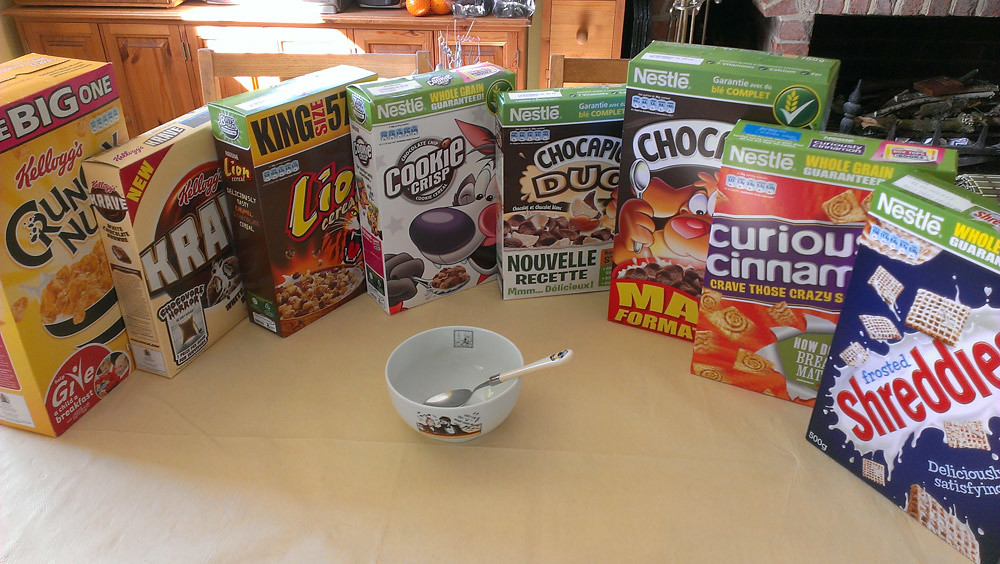This photograph, taken in a kitchen, showcases a diverse selection of breakfast cereal boxes meticulously arranged around a central white bowl with a white-handled spoon. The bowl, featuring a cartoon, sits on a light yellowish-brown table. Surrounding it are eight cereal boxes. Notably, there are Kellogg's Crunchy Nut in a large yellow and red box, Cookie Crisp with a dog on it, and a Nestle Curious Cinnamon box prominently labeled "Crave to Those Crazy." Other boxes include a dark brown cereal box with a tiger labeled King Size, and multiple Nestle boxes topped in green, including a slightly cut-off Frosted Shredded with milk and cereal depicted on it. In the background, brown cabinets and a reddish brick fireplace with neatly stacked wood add to the cozy kitchen setting. This detailed arrangement of cereal boxes presents a colorful and vivid snapshot of a breakfast scene.